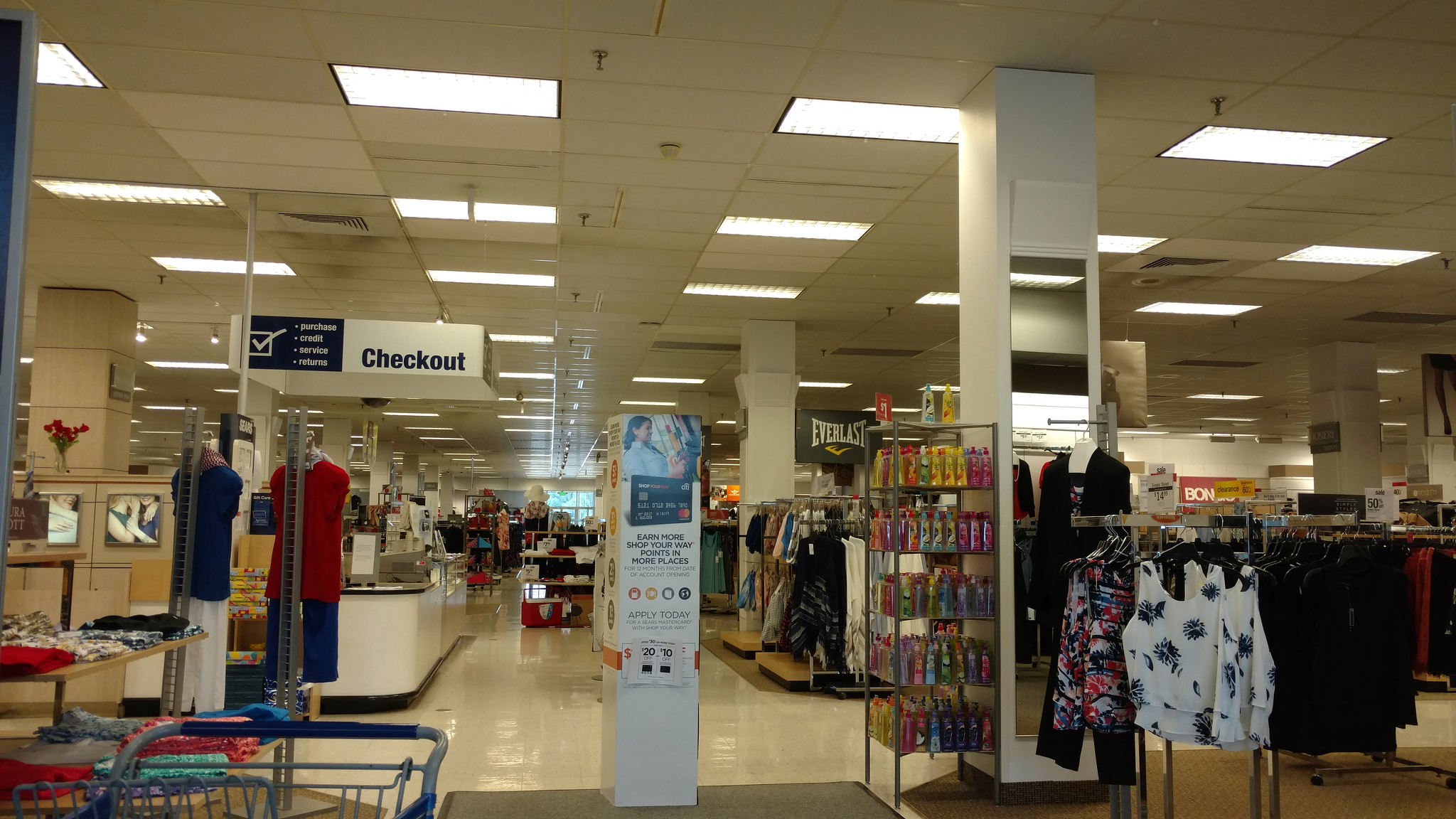The image depicts the interior of a department store, specifically within the clothing and fashion section. The ceiling is lined with commercial-style fluorescent lights, illuminating the space with a bright, even glow. Below, a pristine, white tile floor adds a sleek and clean finish to the environment. To the left of the frame, there is a checkout area featuring a white counter equipped with a cash register, ready to assist customers with their purchases. The store is meticulously organized with numerous clothing racks displaying a wide variety of garments. Toward the center of the image, there's a colorful display of hand soaps and lotions, adding a vibrant touch to the otherwise neutral-toned space. Mirrors are strategically placed on some of the pillars, enhancing the store's spacious feel and allowing customers to check their outfits. The overall atmosphere is orderly and inviting, characteristic of a well-maintained department store.